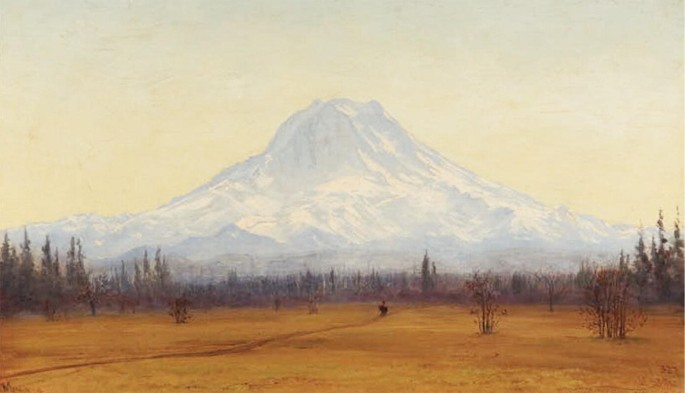The artwork, potentially a painting or a meticulously digitized piece, portrays a vast, almost Wild West scene on a horizontal canvas. Dominating the composition is a trail, a thin, darker brown path cutting through a foreground of golden and lighter brown dirt patches. This trail starts from the lower left and leads towards a diminutive black figure, possibly a person on a horse or a vehicle, far in the distance. The landscape is framed by a mixture of brown and green trees, some crowned with red foliage, standing on either side and converging towards the center of the image. The sky unfolds in a gradient from a foreboding, gray-tinged white to a pale cream at the top. Majestically centered in the background is a colossal mountain, its snow-capped peak painted in shades of white, gray, and light blue, its summit perfectly aligned with the midpoint of the picture. This mountain, coupled with the surrounding scenery, underscores the raw, expansive beauty of the depicted wilderness. The overall color palette consists mainly of neutrals, punctuated by touches of red and blue. In the lower right-hand corner, there's a barely legible artist's signature, possibly accompanied by the numbers "327," adding a personal touch to this evocative and finely executed artwork.